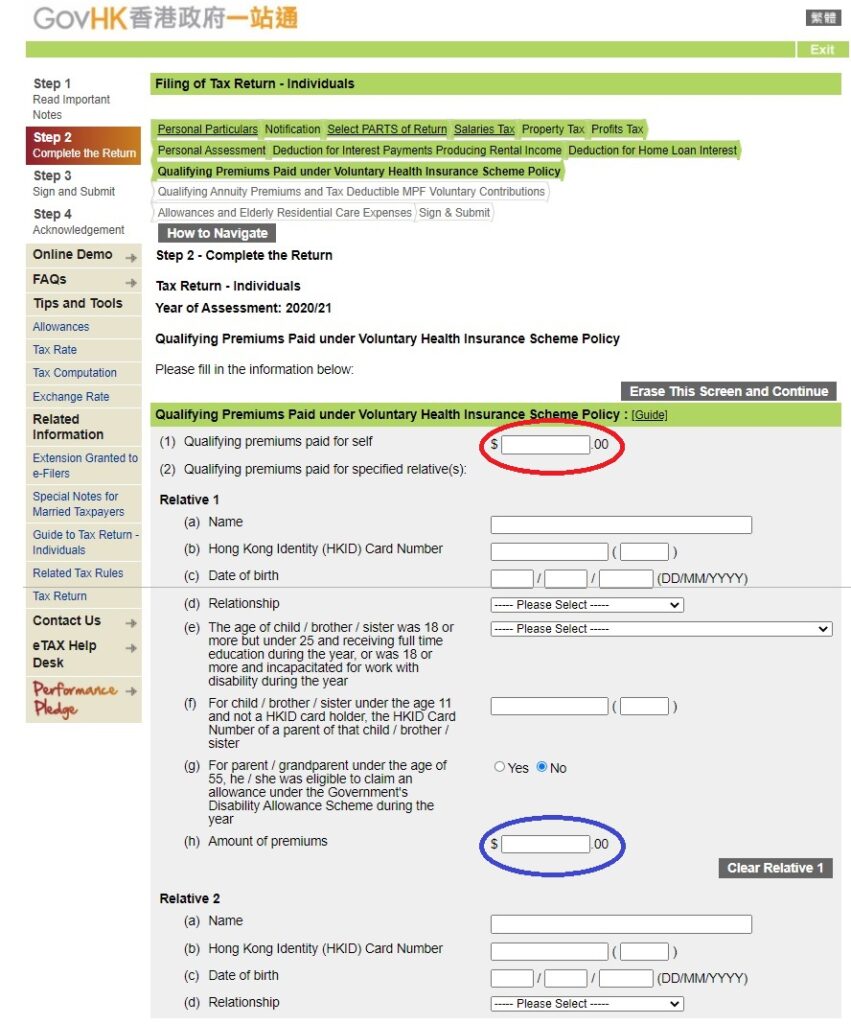Screenshot of a comprehensive website detailing the steps for individuals to file a tax return. The layout is vibrant and utilizes multiple colors including green, red, gray, black, white, and blue. The page is filled with intricate information on completing a tax return. 

On the left-hand side of the screenshot:
- **Step One:** Read important notes.
- **Step Two:** Complete return (highlighted prominently with a red and orange border).
- **Step Three:** Sign and submit.
- **Step Four:** Acknowledgement.

Beneath these steps, additional resources are listed, such as:
- Online demo
- FAQs (Facts and Questions)
- Tips and tools
- Allowances
- Tax rate
- Tax computation
- Exchange rate
- Related information

To the right, under the section "Step Two: Complete the Return", the process of filling out the return form is shown. There’s a specific page dedicated to "Qualifying premiums paid for self," with a significant red circle around a box needing attention. Following that, there are sections for "Qualifying premiums paid for specified relatives" with detailed fields for:
- Relative One: Name, Hong Kong Identity, Date of Birth, Relationship, and Age of the child, brother, or sister.

The entire page appears complex, laden with detailed instructions and numerous fields to fill out, making it challenging to navigate at a glance.